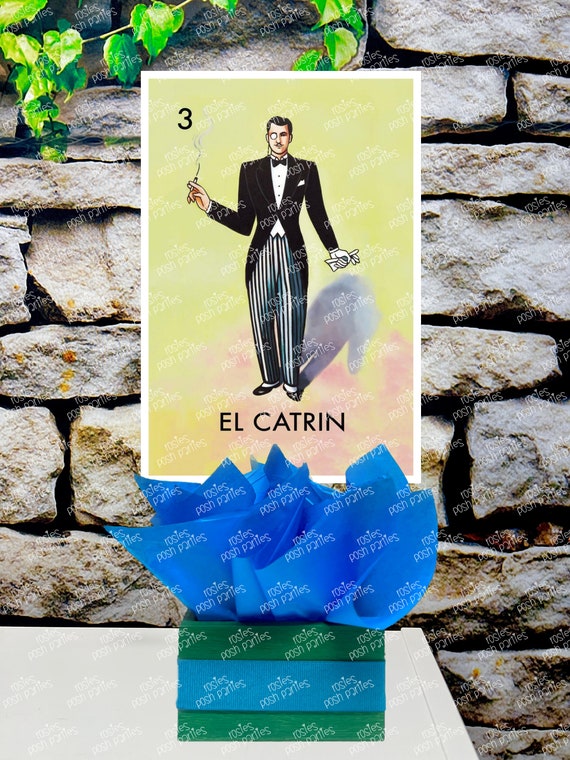The image is a highly detailed drawing of a butler from the 1920s, complete with slick back black hair, a mustache, and a monocle. He is impeccably dressed in a black tuxedo with tails, a white vest, a black bowtie, and black and white striped pants. The butler is holding a cigarette with a cigarette holder in his right hand, and in his left hand, he holds one of his white gloves while the other is worn. The drawing features the text "El Catrin" in black at the bottom and "Rosalie's Posh Parties" in white. This elegant figure is set against a light green background and appears on a card placed atop a green gift box wrapped with a blue ribbon. This assembly sits on a white table, framed by a rustic stone wall adorned with some ivy leaves, adding a touch of nature to the scene.